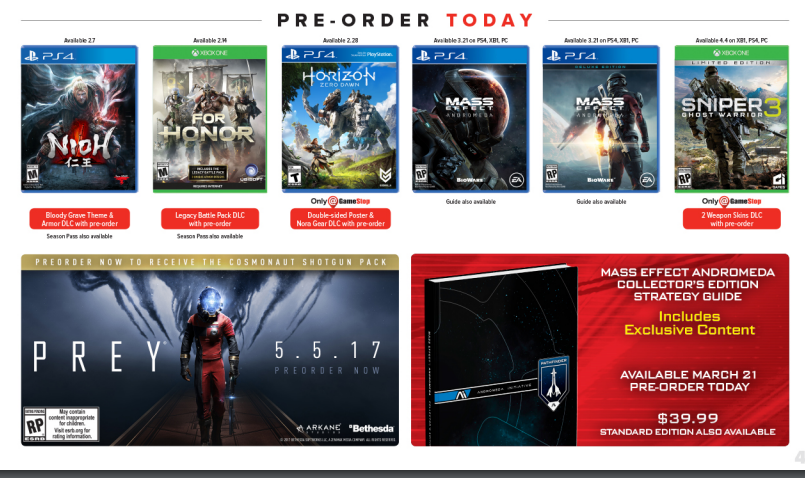The image is a screenshot captured from a computer screen, primarily highlighting a series of pre-order options for various video games. At the top center of the screen, the phrase "PRE-ORDER" is prominently displayed in black font, followed by "TODAY" in striking red, all capital letters. Beneath this header, there is a horizontal row of six images, each showcasing the front cover of a different video game.

From left to right, the first image is of the game "Nioh," which is available on PS4. Next to it is "For Honor," an Xbox game. The third image in the row is "Horizon Zero Dawn," another title for PS4. Following that is "Mass Effect: Andromeda," displayed twice consecutively, with both copies being for PS4. The final image on the right is an Xbox game titled "Sniper Ghost Warrior 3." Underneath the images of the first three games and the last one on the right, there are clickable buttons, suggesting access to more information or purchase options.

On the left side, beneath the row of video game covers, is an advertisement for the Bethesda game called "Prey," which lists its release date as 5-5-17. The ad urges readers to "Pre-order Now," and includes a warning label in the bottom left corner. Adjacent to this, on the right side, is another advertisement with a vibrant red background. This ad features a black book adorned with a spaceship logo and the title "Mass Effect: Andromeda Collector's Edition Strategy Guide." This guide includes exclusive content and is available from March 21 for $39.99, with a note that a standard edition is also available.